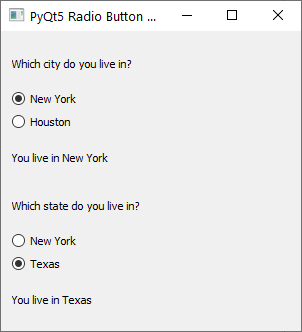This image appears to be a partial screenshot of a website interface, specifically focusing on the upper section. 

### Upper Section:
- **Banner (Upper Left):** Spanning the entire width of the image, the banner features a notable white paper icon with blue details and a small, dark gray line at the top.
 
### Upper Right Hand Side:
- **Label:** Adjacent to the icon, text reads "PyQt5" with a radio button to its right, followed by a space, a hyphen, another space, a square, and an "X."

### Middle Section:
- **Grayed-out Area (Questionnaire):** Beneath the banner, there's a gray section containing interactive content.
  - **Question:** "Which city do you live in?"
  - **Options:** 
    - "New York" (highlighted in black)
    - "Houston" (with an unselected white circle)

### Bottom Section:
- **Selection Display:** The text "You live in New York" is displayed, followed by another gray space.

- **Question:** "Which state do you live in?"
  - **Options:**
    - "New York" (with an unselected white circle)
    - "Texas" (with a selected, black-filled circle)

- **Selection Display:** The text "You live in Texas" is shown underneath.

This descriptive breakdown captures the elements and layout of the image, providing a clear understanding of its content.